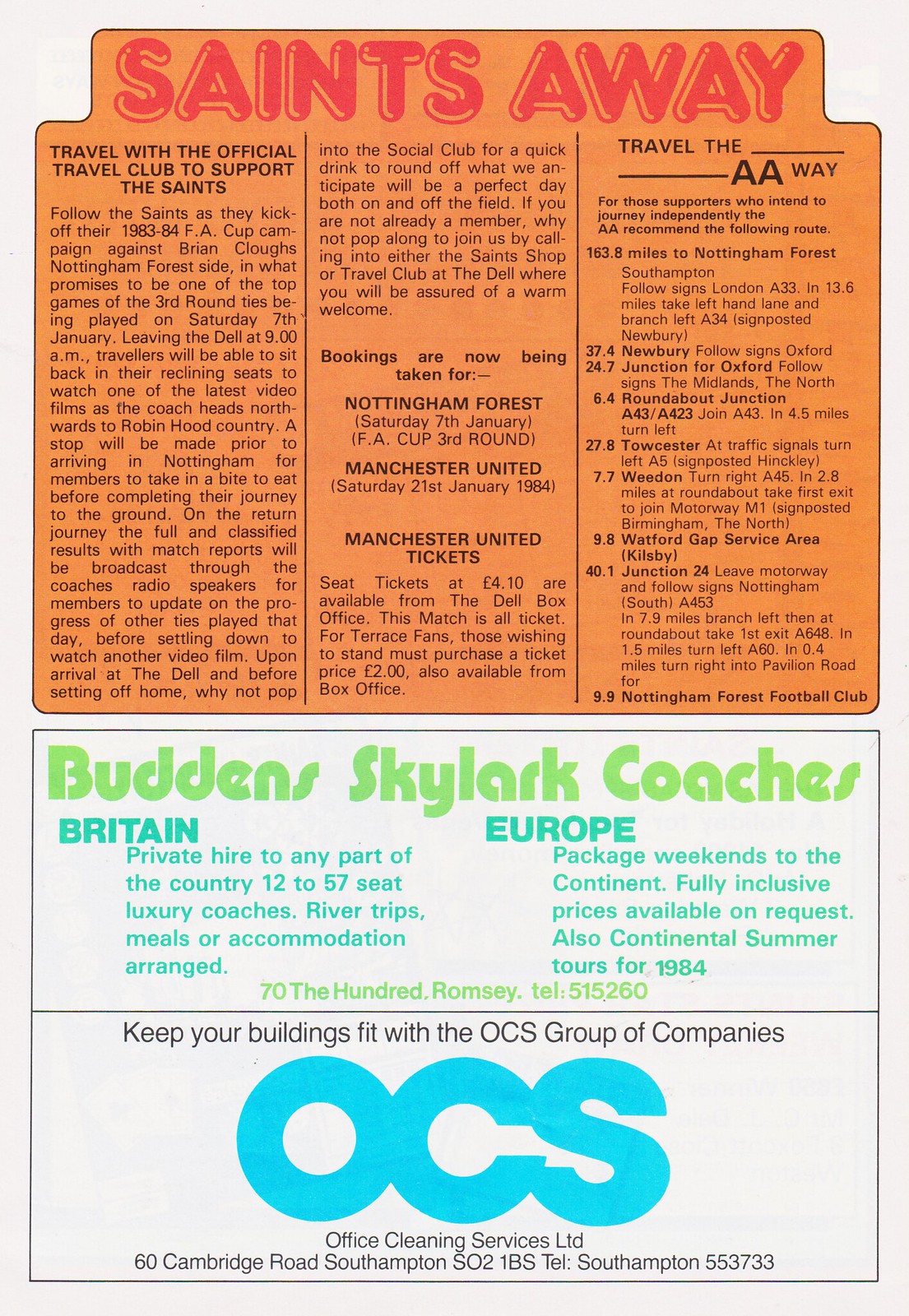The image is a rectangular news article measuring about six inches tall and four inches wide, featuring a light gray border encasing two main sections, each with a thin black border. The top section has an orange background and prominently displays the title "Saints Away" in bold orange letters with a light orange shadow. Beneath this, there are three columns of text. The left column is titled "Travel with the Official Travel Club to Support the Saints," inviting fans to join the Saints' official travel club as they embark on the 1983-1984 FA Cup campaign. The center column mentions that bookings are now being taken for upcoming matches against Nottingham Forest and Manchester United, with specific mention of tickets for these games. The right column states "Travel the AA Way," with a blank line interspersed, followed by sections detailing various travel options.

The bottom section is divided horizontally into two parts. The upper part features a green rectangle with the inscription "Bud and Skylark Coaches" and lists "Britain" and "Europe" in blue text. Below it, there is contact information in light green text: "7100 Romsey Telephone 515260." The lower part includes another black-bordered rectangle advertising "Kiefer Buildings" in collaboration with the OCS Group of Companies, listing their services and contact details: "OCS - Office of Cleaning Services, LTD, 60 Cambridge Road, Southampton, SO2, 1BS, Telephone Southampton 553733." The article highlights the journey to the Saints' FA Cup third-round match against Nottingham Forest on Saturday, January 7th, detailing the amenities provided during travel, such as reclining seats, in-coach video films, meal stops, and broadcasted match reports.